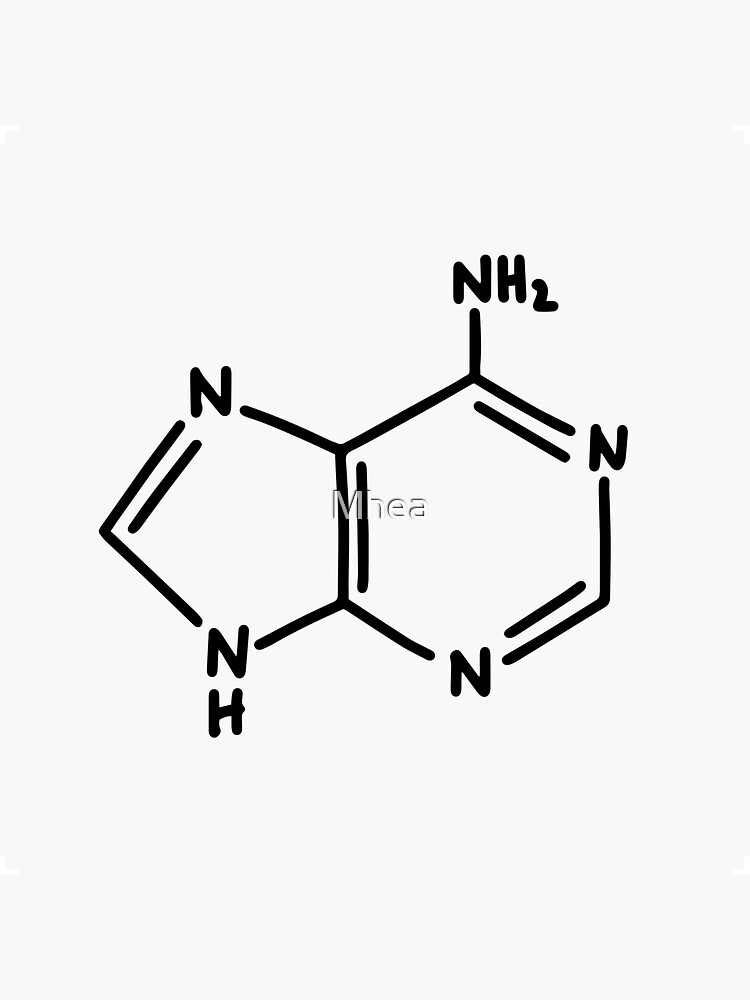The image showcases a detailed structural diagram of a chemical molecule, composed of a pentagon joined to a hexagon on the right. The pentagon on the left features a nitrogen (N) atom at the top and an NH group at the bottom. The adjoining hexagon on the right displays an NH2 group at the top, another nitrogen (N) atom on the top right corner, and additional nitrogen (N) atoms at both the bottom right and bottom corners. Some sides of the shapes reveal extra lines that signify double bonds. The diagram is presented in black lines and letters set against a slightly off-white background, giving it a hand-drawn appearance. Additionally, the word "MHEA" appears superimposed over the diagram.